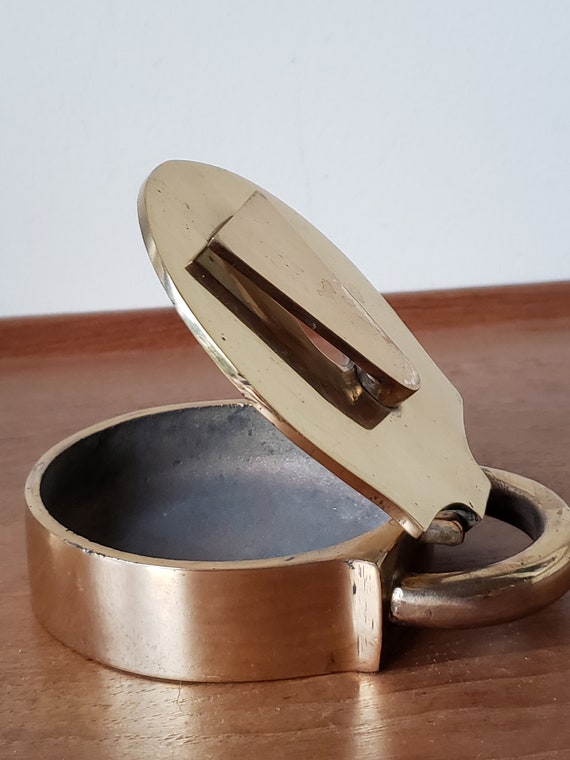This close-up photograph showcases a unique, bronze-like lock resting on a medium-stained wooden surface, with a plain white wall in the background. The central object resembles a locket or padlock and is goldish-bronze in color, with a shiny, muted metallic finish. The lock is open, revealing a hollowed interior that is tarnished black. The lock features a top lid and a bottom half, with a small lever on the top lid that likely assists in opening and closing the mechanism. Perched on the top is a metal hook or handle designed for hanging. Additionally, there is a metal triangular piece attached to the lid, which is propped open, showcasing the square, bowl-like interior. The detailed craftsmanship and unique functionality draw your eyes directly to this intriguing metallic object.